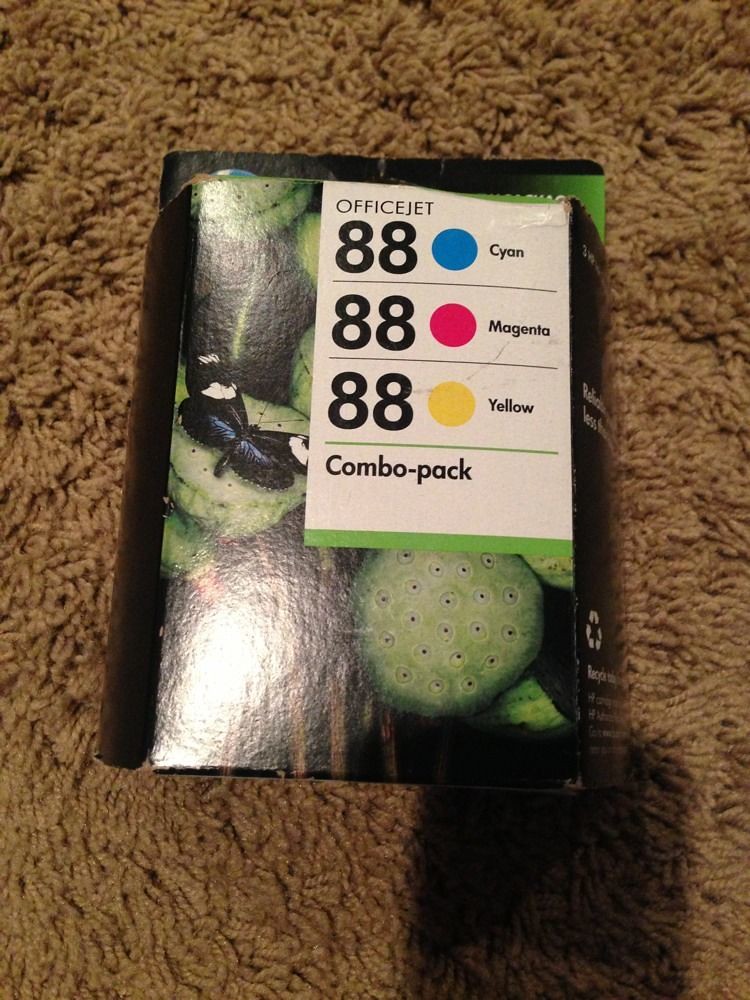The photograph shows a slightly battered box of OfficeJet printer ink cartridges lying on a matted brown shag carpet. The box, primarily in shades of green and black, displays a blurred color photograph of a purple-black butterfly with white spots perched on a cactus bud. A clear shadow of the phone used to take the picture is visible in the lower right corner. In the upper right quadrant of the box is a detailed label: "OfficeJet Combo Pack" in black text. There are circular color indicators next to the number "88" – a blue circle for cyan, a pink circle for magenta, and a yellow circle for yellow. The combo pack's glossy paper package is slightly crushed and reflects a blown-out overhead light, adding to the worn appearance. A recycling logo and additional text are present on the side of the box.